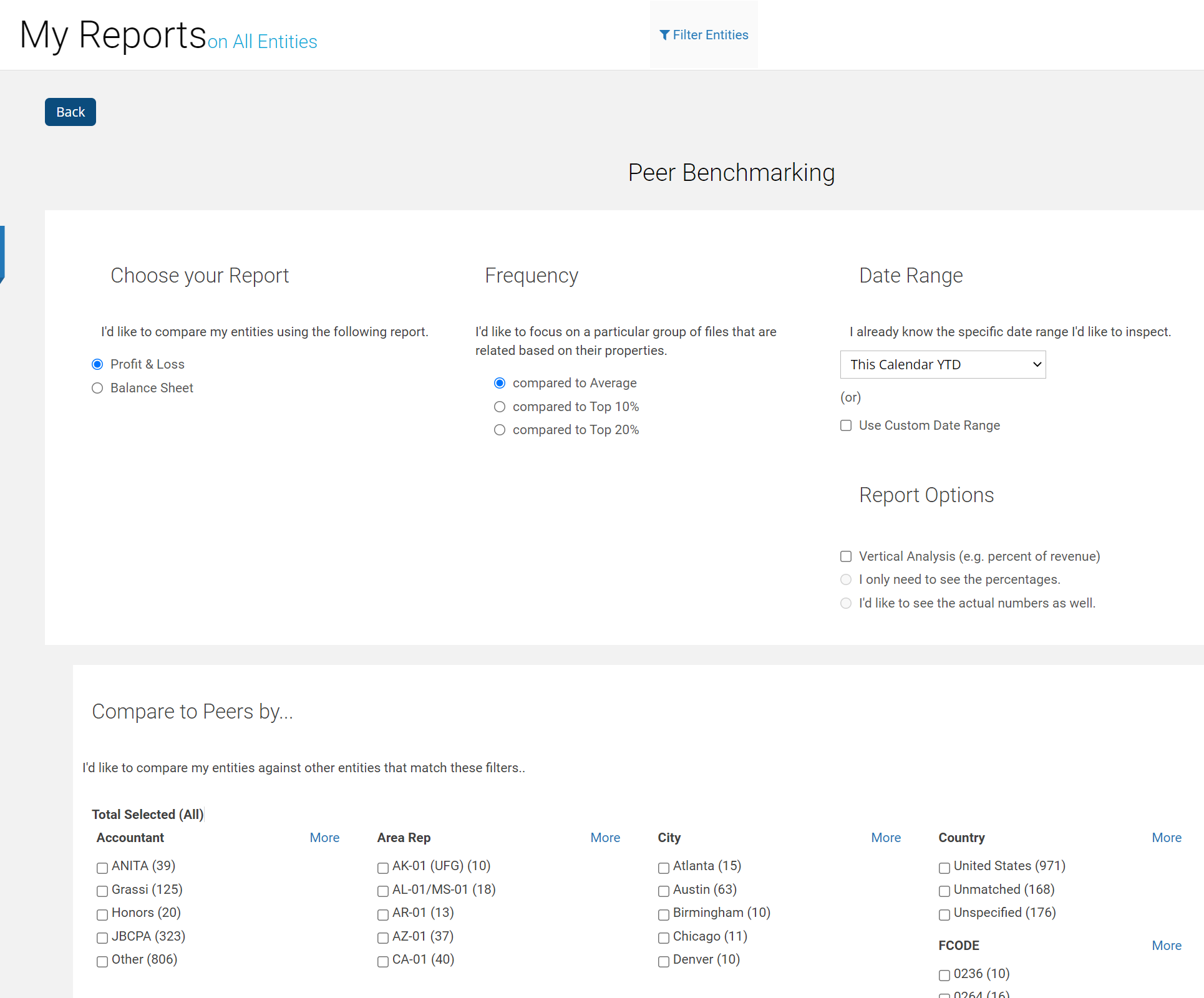Here is a detail-oriented and polished caption for the screenshot described:

"This screenshot, labeled 'My Reports,' is divided into two main sections. The first section is titled 'Peer Benchmarking,' prominently displayed above a white box that contains four distinct subsections. 

The first subsection, 'Choose Your Report,' offers two options: 'Profit and Loss,' which is selected and highlighted in blue.

The second subsection, 'Frequency,' provides three choices, with 'Compared to Average' selected and highlighted in blue at the top of the list.

The third subsection, 'Date Range,' features a drop-down menu and a checkbox for 'Use Custom Date Range,' though no options are currently selected.

The fourth subsection, 'Report Options,' includes three items: a checkbox labeled 'Vertical Analysis' and two further options displayed as radio buttons.

Adjacent to this is the second section, titled 'Compared to Peers By.' This section is broken down into five categories:

1. 'Accountant' – featuring approximately five options.
2. 'Area Rep' – also featuring about five options.
3. 'City' – listing specific cities such as Atlanta, Austin, Birmingham, Chicago, and Denver.
4. 'Country' – with 'United States,' 'Unmatched,' and 'Unspecified' as options.
5. 'F Code' – offering two options.

Each category in the 'Compared to Peers By' section includes a 'More' link on its right side, presumably for additional options."

This caption provides a thorough and precise description of the contents of the screenshot, making it easy for someone to visualize the layout and options available.